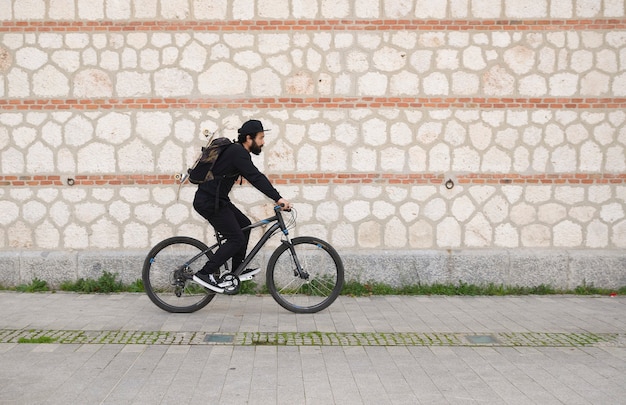In the image, a man is riding a black mountain bike on a brick or stone pavement. He is dressed entirely in black, wearing a black long-sleeve shirt, black pants, a black baseball cap, and black and white tennis shoes. His outfit is complemented by a black and brown backpack, which appears to have a skateboard mounted on it. The man has black hair and a black beard.

The pavement beneath him includes a strip of older-looking stones with grass or moss growing between the cracks, and there's a drainage grate running along it. Behind him stands a distinctive white stone wall featuring four broad rows of slightly pinkish, giant pebble-like stones. These rows are separated by narrow stripes composed of two layers of red bricks. The base of the wall has very green weeds sprouting where it meets a tall curb. The scene provides a strong visual contrast with the man's dark attire against the textured backdrop of the pavement and stone wall.